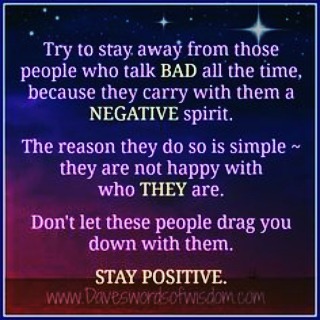The image looks like a digital poster or clip art from the internet and is sourced from www.daveswordofwisdom.com. The background transitions beautifully from dark starry skies in black, through purples, to deep blues, magentas, and reds from top to bottom. A white line border frames the aesthetically pleasing scene. The text is a motivational message written mostly in purple with certain words highlighted in tan for emphasis.

At the top section, the text reads: "Try to stay away from those people who talk bad all the time because they carry with them a negative spirit." The words ‘BAD’ and ‘NEGATIVE’ are in uppercase and tan to emphasize the cautionary note. 

In the middle section, the background shifts to a dark blue as the message continues: "The reason they do so is simple. They are not happy with who they are." Here, the word ‘they’ is also capitalized and tan, drawing attention to the source of negativity.

Towards the bottom, against a deep red background, the concluding advice reads: "Don't let these people drag you down with them. Stay positive." The phrase ‘STAY POSITIVE’ is in uppercase and tan, underscoring the importance of maintaining a positive mindset.

At the very bottom of the image, the website www.daveswordofwisdom.com is subtly included, suggesting the source. This motivational poster features a harmonious blend of colors and carefully chosen emphatic words, making it a wonderful piece for inspiration and positive reinforcement.